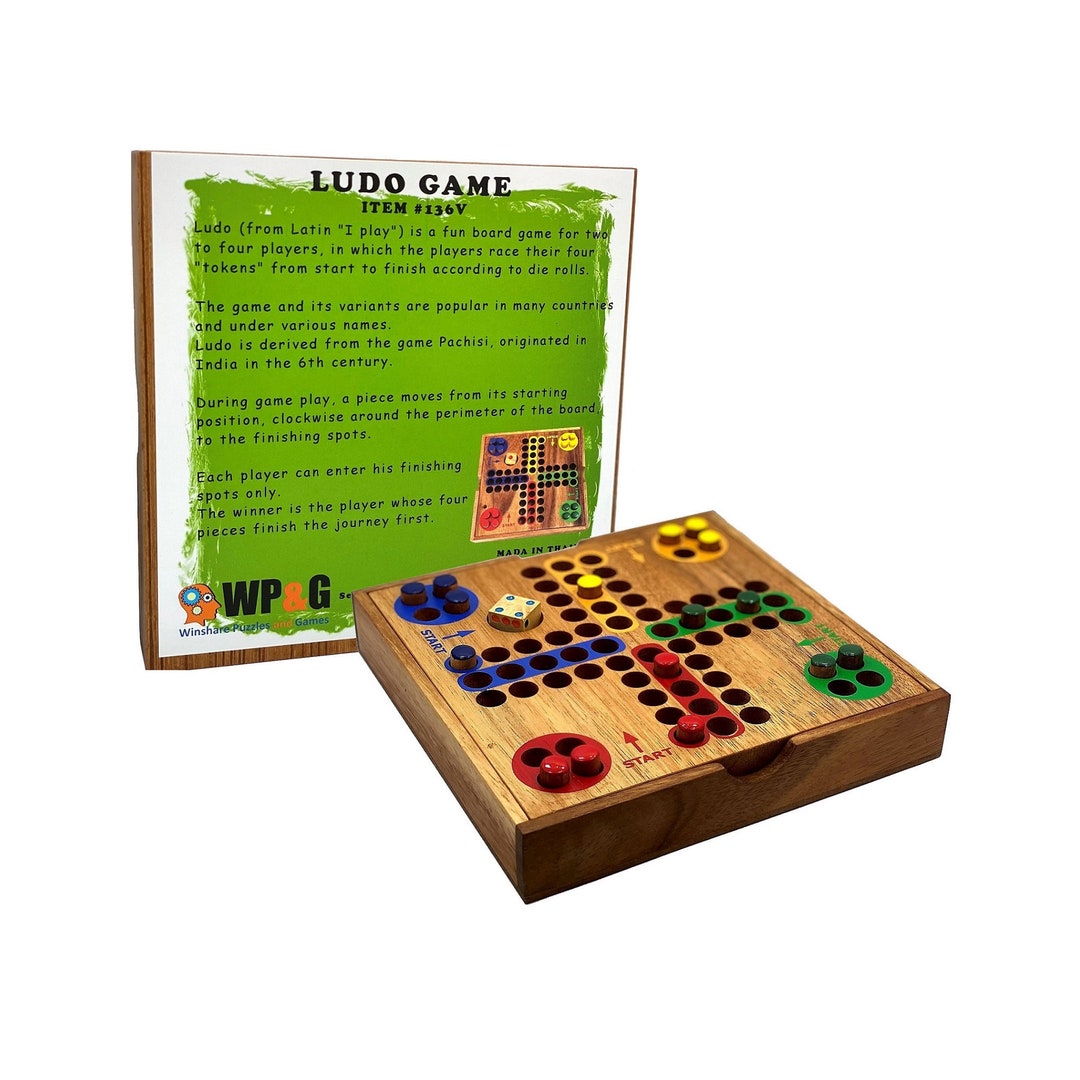This detailed image depicts a wooden Ludo board game. The board features a cross in the center created with rows of tiny holes: the top arm of the cross is yellow, the left arm is blue, the bottom arm is red, and the right arm is green. Each arm consists of three rows of holes, making a total of 12 rows on the board. At the corners of the game board are four circles, each color-coded to correspond with the arms of the cross: the top corner is blue, the right corner is green, the bottom corner is red, and the left corner is yellow. Within these circles, there are recesses to hold up to four game pieces, though some colors don't have all four pieces present. 

Accompanying the game board, standing upright, is a poster stating 'Ludo Game' (spelled L-U-D-O). It details the rules and origins of the game: Ludo, derived from the Latin "I play," is a classic board game for 2 to 4 players. The goal is for players to race their four tokens from start to finish based on die rolls. The description notes that Ludo is derived from the ancient Indian game Pachisi, popular worldwide under various names. The instruction sheet further explains the movement of pieces clockwise around the board and how the game concludes when a player's four tokens finish their journey first.

The board seems to have a storage space below, as it's described as a box, hinting that parts can be stored underneath the playing surface. The image also shows a die near the board, essential for gameplay. Item number 136B signifies this particular Ludo set.